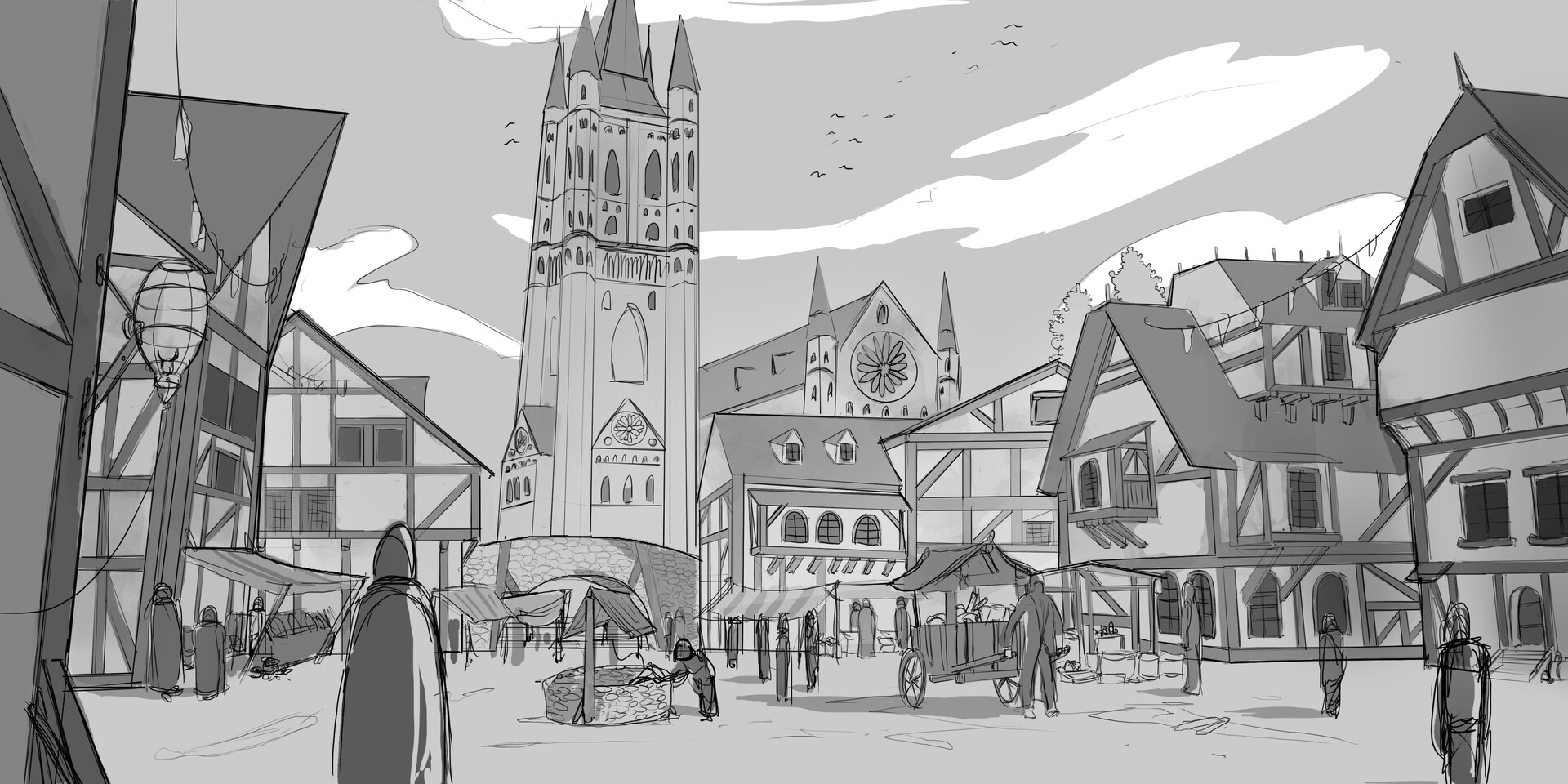In this cartoon-style drawing, a quaint European town from yesteryear is vividly depicted. The scene centers around a collection of charming, gray-toned buildings adorned with intricate wooden trim, exuding a Scandinavian flair. Dominating the background is an imposing, slender castle, characterized by its numerous spire-like points. The sky overhead is a muted gray, speckled with fluffy white clouds, adding a somber ambiance to the illustration. In the foreground, a woman draped in a flowing gray cloak that covers her head stands prominently. Near her, a person is bent over a large well, while a small cart sits nearby, suggesting a bustling life in this serene, historical setting.